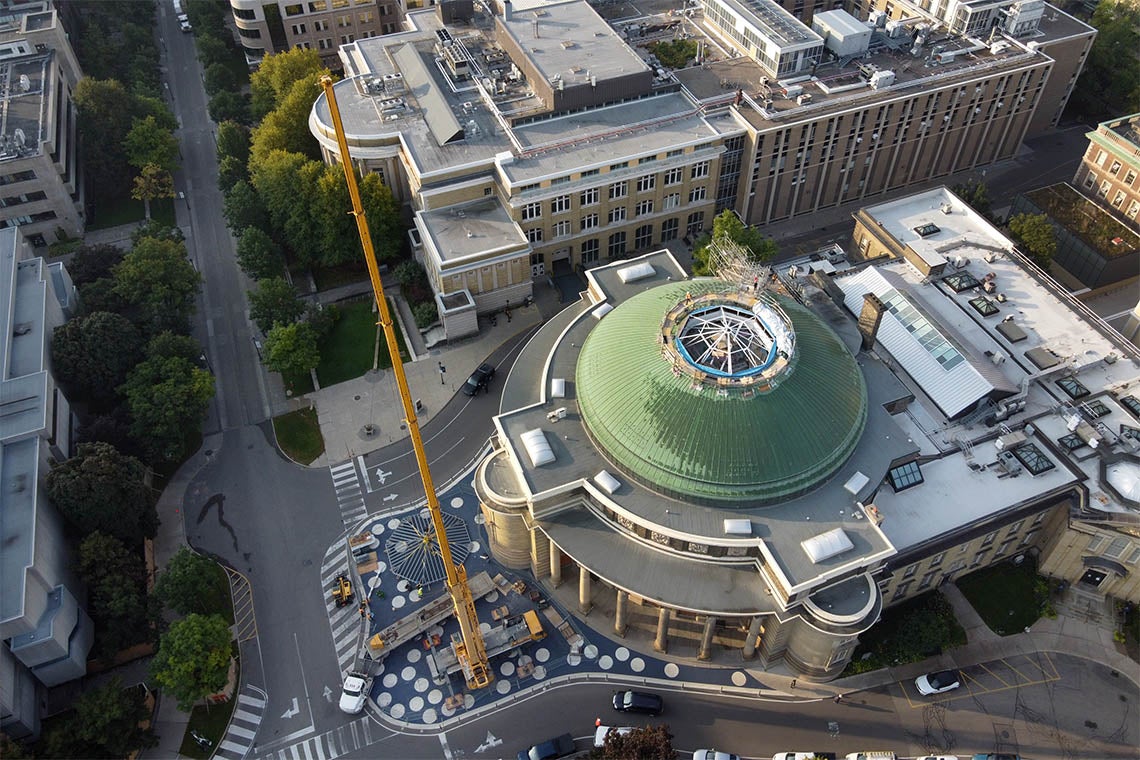An aerial view of a downtown area captures two prominent buildings as the main focal points. The forefront features a distinct building with a green dome-like portion on its roof and classical columns on its semi-circular front section, clearly marked by a yellow crane indicating ongoing construction work. Directly in front of this structure, a street runs vertically from top to bottom, separating it from another significant tan building behind it. This building, characterized by numerous windows, sits amidst a cluster of trees and has a road running in front of it. Additional details reveal cars moving along the roads that interweave between these buildings, and some construction equipment is seen scattered within the vicinity of the domed building, including a blue area dotted with white circles, adding to the bustling ambiance of the urban landscape. To the left edge of the photograph, more buildings and greenery add depth to the city's dynamic environment.